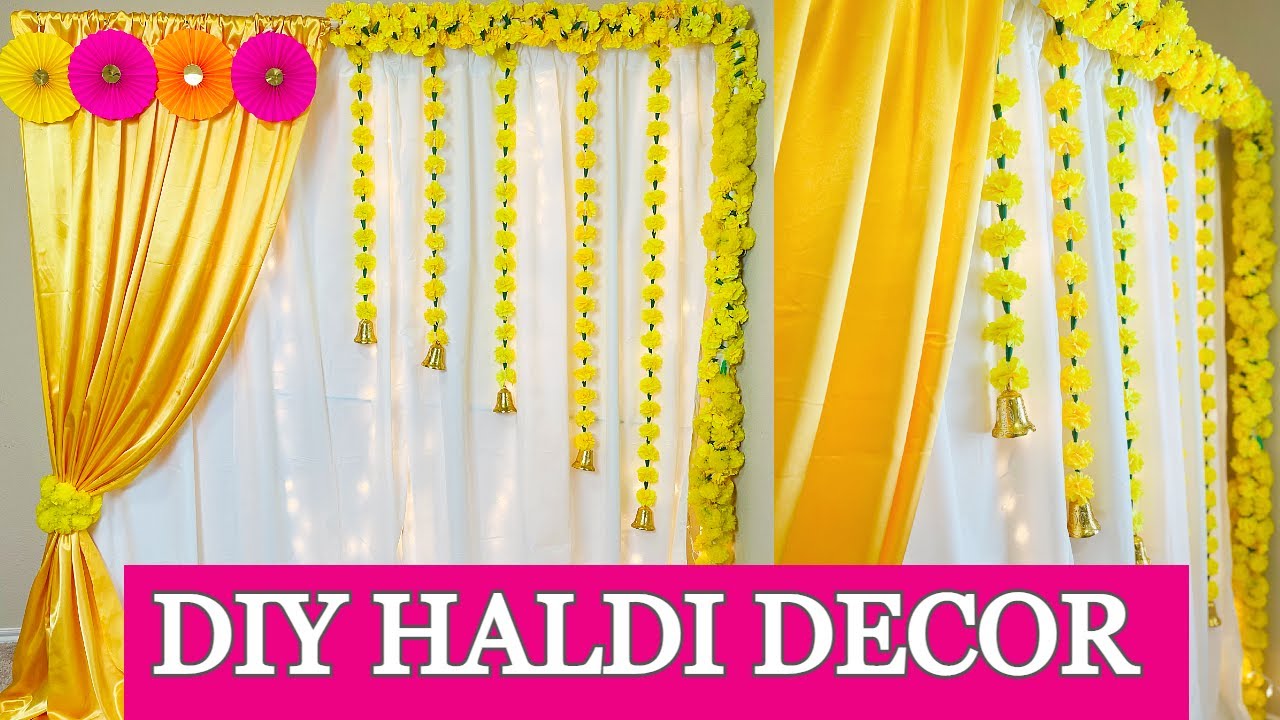The photograph showcases an intricate DIY Haldi decor setup, prominently featuring golden satin or silk curtains adorned with paper flowers and floral decals. At the top of the curtains, four circular fans in yellow, pink, orange, and pink colors add a splash of vibrancy. Strands of yellow flowers, each ending with a gold bell, hang down from green strings, creating a cascading effect. The left side of the image shows the golden curtain tied with a decorative element near the bottom, while the right side provides a close-up, angled view of this arrangement. Overlaying the image is a large pink banner with white capital letters that read "DIY Haldi Decor". Various angles of the curtain decorations are combined to offer a comprehensive view of the setup, emphasizing its elegance and festive spirit designed for a Haldi ceremony.